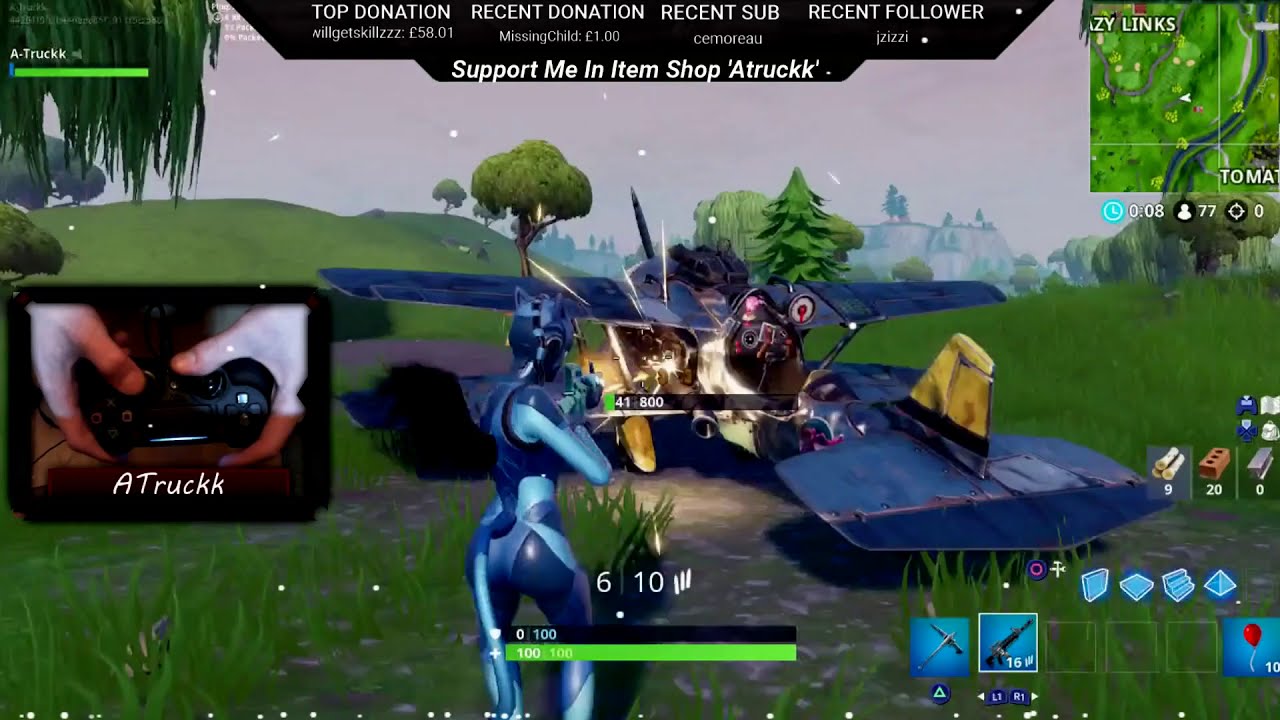In this detailed scene from a video game livestream, a female player is shown on the left side of the screen holding a game controller. Dominating the center of the screen is the game itself, depicting a blue, feline-like fantasy character reminiscent of a figure from "Avatar." This character, equipped with a gun, is actively shooting at a blue and yellow vintage propeller plane that has landed on a grassy field. The background features lush greenery, trees, rolling hills, and distant mountains, enhancing the fantasy setting. The stream interface includes various overlays: at the top are labels for "top donation," "recent donation," "recent sub," and "support me." A minimap is situated in the top right corner, displaying the game area, and inventory details appear at the bottom right. The streamer, identified by the username A-Trek, provides his viewers with a real-time view of his hand positioning on the controller to improve engagement. This vibrant scene is accentuated by a mix of green and blue hues, highlighting the fantastical and immersive nature of the game, which resembles "Fortnite."